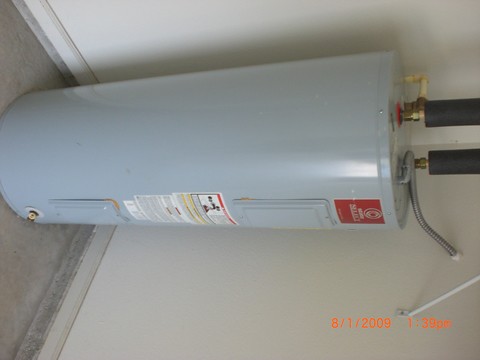This sideways color photograph, date-stamped "8-1-2009 1:38 p.m." in the bottom right corner, features a gray cylindrical hot water heater positioned on a cement floor. The white walls surrounding the heater indicate it is located in a corner. The hot water heater bears several stickers. At the top of the heater, a copper pipe, wrapped in black tape, is visible. Additionally, a silver metal tube extends from the side of the heater into the wall.